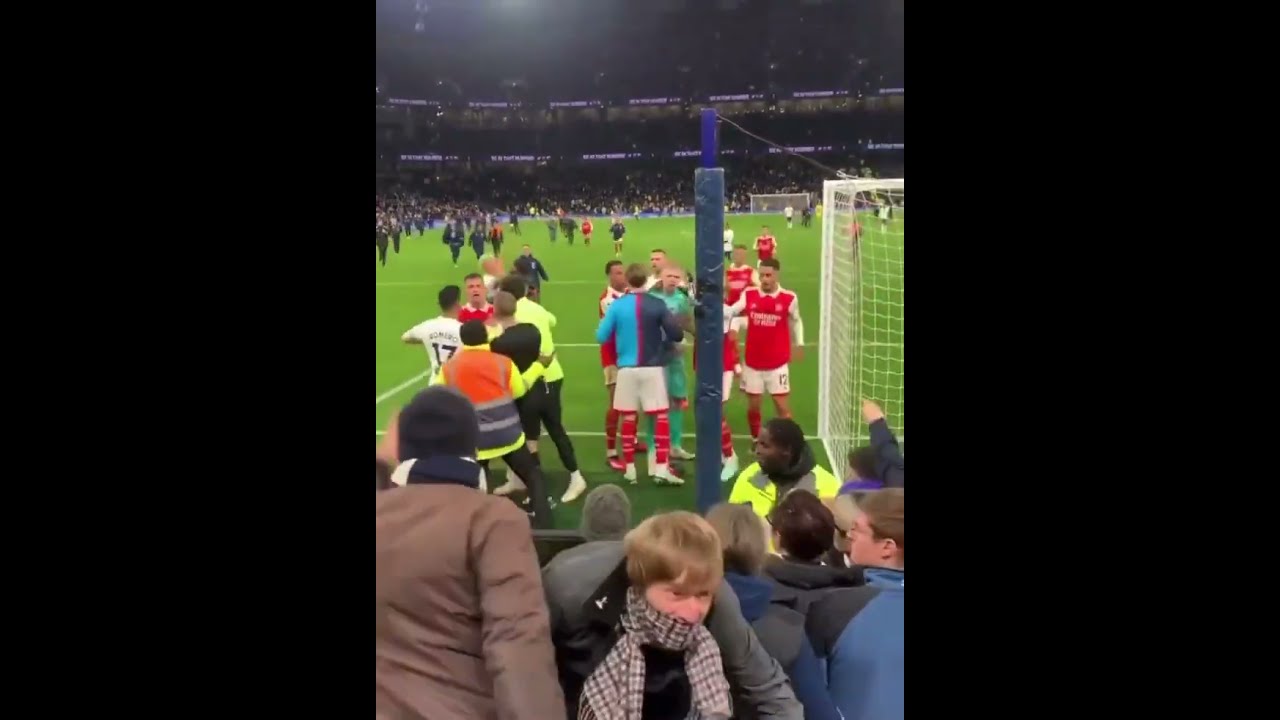The image captures a chaotic scene taking place at a nighttime soccer match in a large, well-lit stadium. The photograph is taken from a vantage point behind one of the goalposts, with the net visible to the right. Players in red and white uniforms are congregated near the goal, appearing to be in a heated discussion or argument. Opposite them, individuals in green uniforms are being held back by a man dressed in red socks, white shorts, and a blue two-toned top. Another cluster of red-uniformed players on the left side of the image is being restrained by people in black pants and yellow shirts. The foreground of the image shows the audience, with one notable figure wearing a gray shirt and a checkered scarf around his face, looking towards the action as if surprised or concerned. The field is green, and despite the apparent conflict, no one is violently clashing, hinting at confusion rather than a full-blown riot. The sides of the photograph are outlined with a thick black border, framing the otherwise vibrant and animated scene.